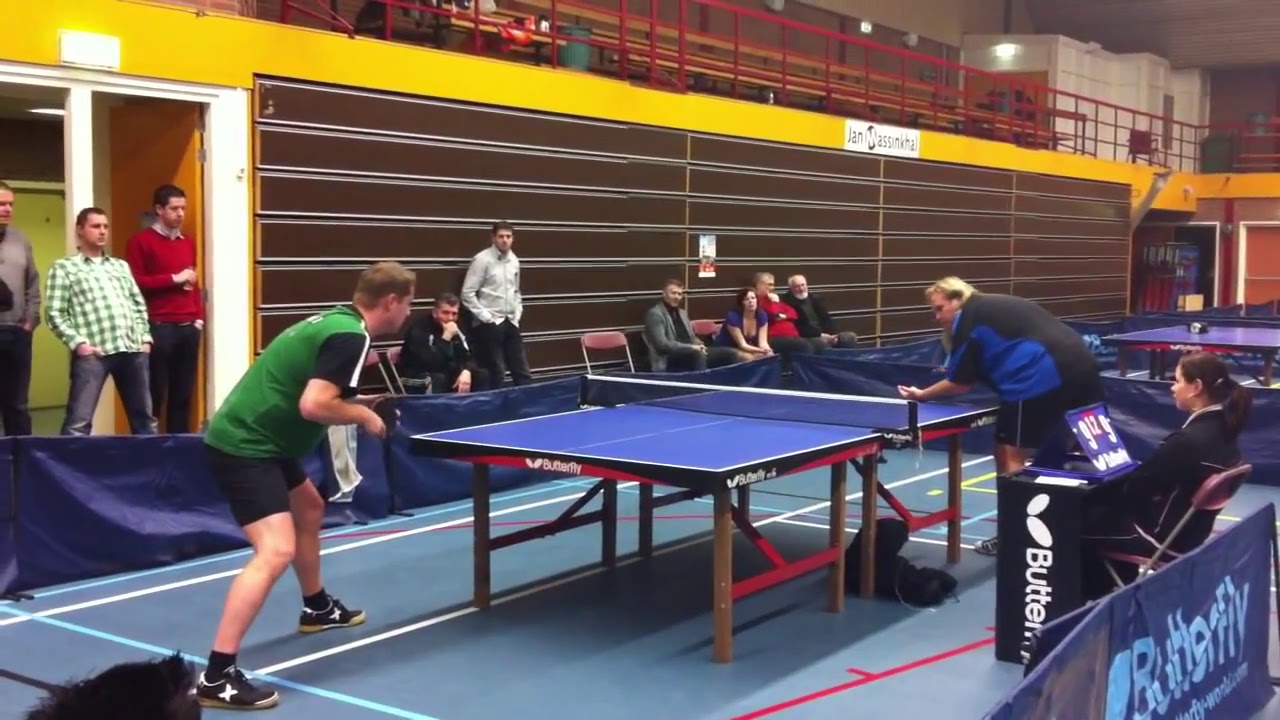The image captures a lively scene of a ping-pong tournament taking place in a large gym-like space, possibly an arena. The blue ping-pong table is central to the composition, around which the match unfolds. On the left side of the frame, a man in a green and black shirt, black shorts, and black shoes is poised to hit the ball. Opposing him, a heavyset blonde woman, wearing a blue and black shirt and black shorts, leans over the table, holding the ball in her left hand, seemingly ready to serve.

The gym features an upstairs area with a distinctive red railing, which might be a running track. To the right of the ping-pong table, a woman dressed in black sits at a smaller table with a flip scoreboard displaying the score. The scoreboard has a Butterfly logo on it, indicating official tournament equipment.

A sizable audience, comprising both seated and standing spectators, can be seen to the left side and in the background, showing keen interest in the competitive match. Their presence reinforces the ambiance of an official and organized sporting event.